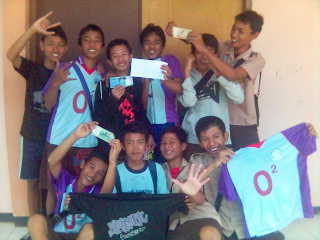This somewhat out-of-focus and small photograph appears to be an older image, featuring a group of nine boys with tan, darker complexions who are visibly happy and posing for the camera. They are dressed in summertime clothing, predominantly in white and purple t-shirts, with some variations in red, black, and blue. The boys are arranged in two rows: five standing in the back and four squatting in front. They are holding various items including t-shirts, pieces of paper, and money, and they seem to be celebrating, possibly having just won something. A noticeable detail on the jerseys is the number '0' with a squared symbol on the right side. Despite the poor photo quality, their cheerful expressions and gestures, such as thumbs up and rock on signs, suggest a joyful event, possibly a school or community gathering, with the background featuring a white wall.